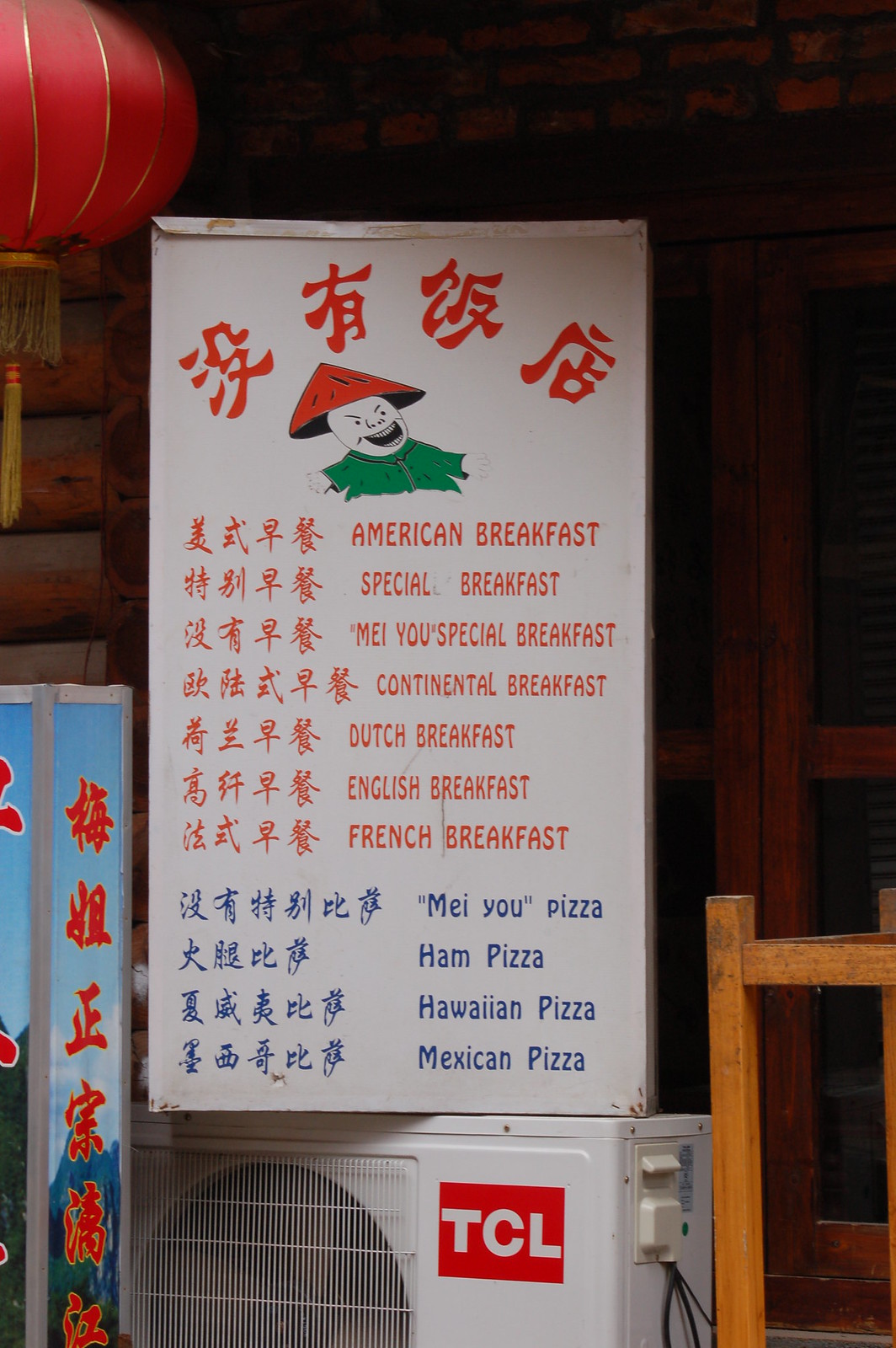The image showcases a prominent white sign situated in front of a restaurant. The sign features vibrant orange text, primarily in a language other than English. At the top of the sign, there is an illustration of a smiling character with a somewhat whimsical appearance, wearing an orange, pointed triangular hat and a green shirt. Below this cheerful figure, additional orange text in a foreign language is visible, reinforcing the international flair of the establishment. Amidst the foreign script, several English phrases are prominently listed, advertising a variety of breakfast options and pizzas available at the restaurant. The English phrases include "American Breakfast," "Special Breakfast," "My You Special Breakfast," "Continental Breakfast," "Dutch Breakfast," "English Breakfast," "French Breakfast," "Me You Pizza," "Ham Pizza," "Hawaiian Pizza," and "Mexican Pizza."